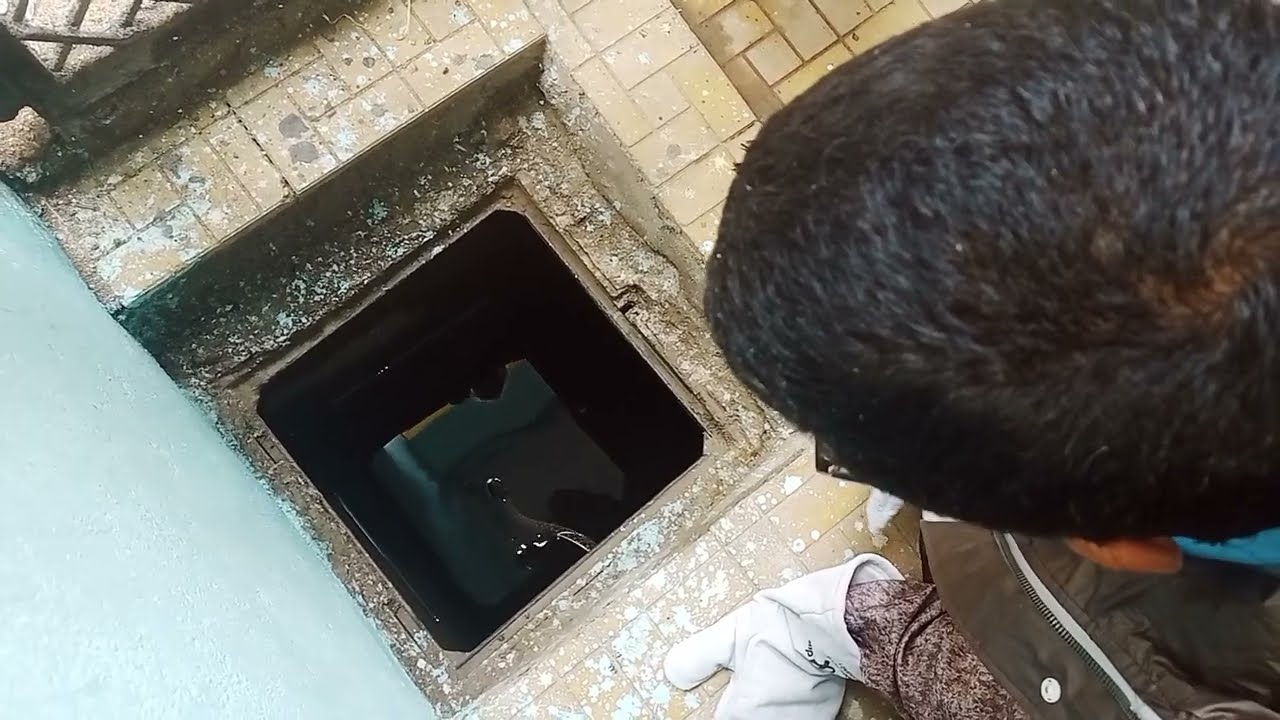The image shows a man with short, black hair and glasses, focused intently downward into a murky, dark area below. He's wearing a brown vest over a shirt, with long sleeves, and has a white glove on his left hand. The man is either kneeling or on his hands and knees, appearing to be working on or inspecting something that resembles a drain or an open square hole. Tilings surround the hole, creating a stepped effect, with a blue surface visible to the bottom left and concrete to the upper left. The scene is detailed with different textures, indicating it is three layers deep below the surface.